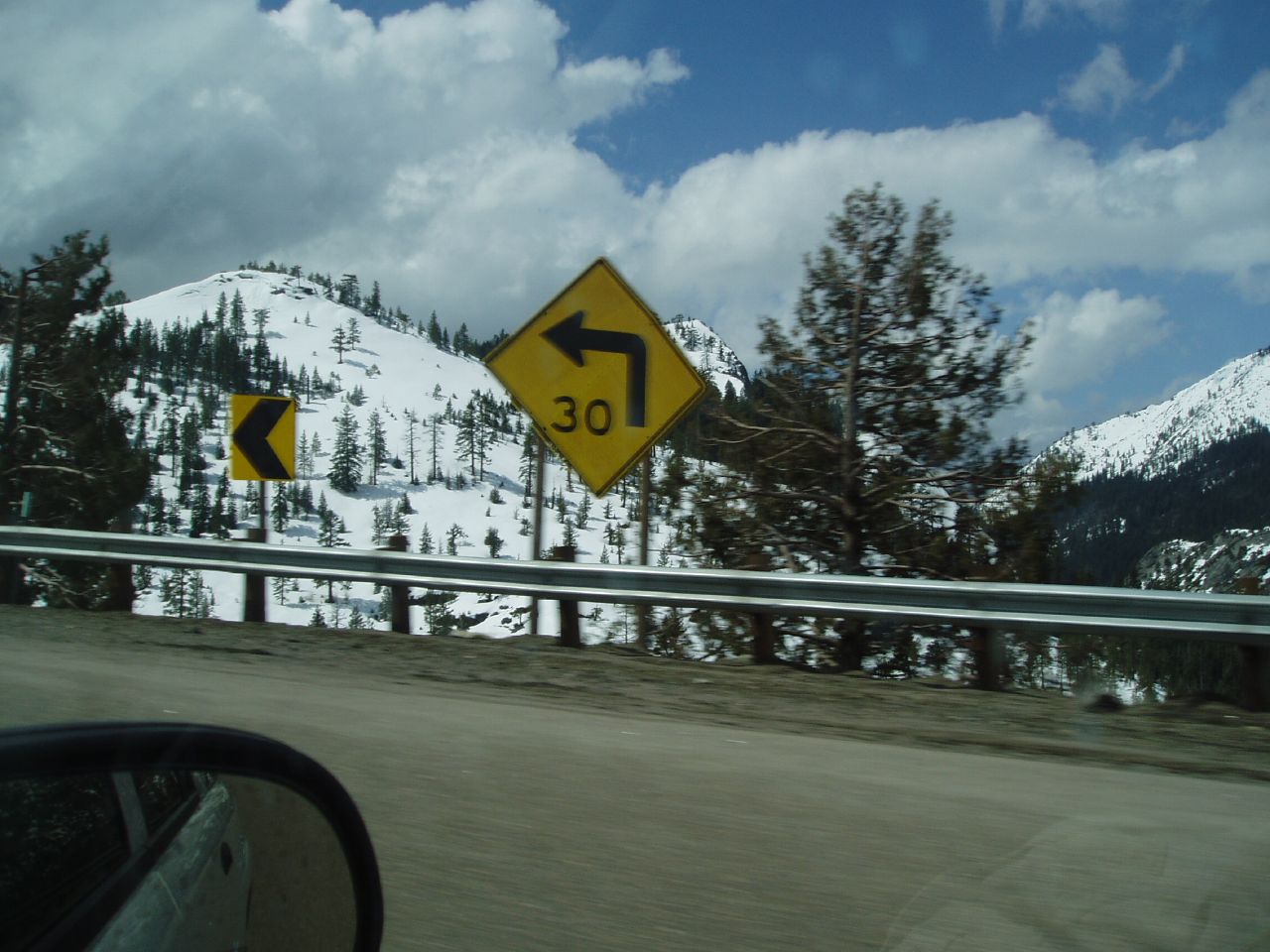The photograph captures a scene from the passenger side of a moving car, showcasing a striking mountainous landscape. The car's side mirror, reflecting part of a blue midsize sedan, indicates the image is taken from the vehicle's right side. Prominently featured in the foreground are two yellow road signs mounted above a sturdy, silver guardrail supported by short black posts. The primary sign is a diamond shape with a black right-angle arrow pointing left, accompanied by the number '30,' though no unit of measure is specified. Adjacent to it is a smaller rectangular yellow sign with a black arrow pointing left.

Beyond the guardrail, the scene expands to reveal majestic, snow-covered mountains that rise to sharp peaks, reminiscent of ski slopes. Some areas of the mountains are densely populated with evergreen trees, while others are sparsely vegetated. The sky overhead is a brilliant blue, scattered with large, fluffy white clouds, suggesting it's a bright, sunny day. The detailed layers of snow enveloping the mountains and the contrasting palm trees create a striking and somewhat surreal visual juxtaposition.